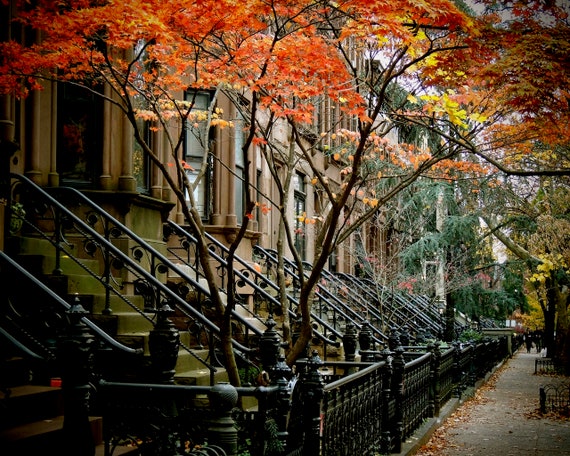The image showcases a quintessential New York City street in the fall, characterized by a row of iconic brownstone houses. The brownstones display varying shades of tans and browns with a uniform architectural style, featuring cement stairs leading up to the doorways, and distinctive windows, each with three sets of individual panes that slightly protrude out. The black wrought iron railings and fences surrounding the front of each building and the trees lining the street contribute to the classic cityscape. The trees, some enclosed by black metal fences, are in full autumn splendor with leaves turning vibrant hues of red, yellow, and orange. Scattered leaves blanket the cobblestone-lined sidewalk, adding to the seasonal ambiance. In the distance, people are seen walking, enhancing the lively urban atmosphere of this picturesque fall scene.